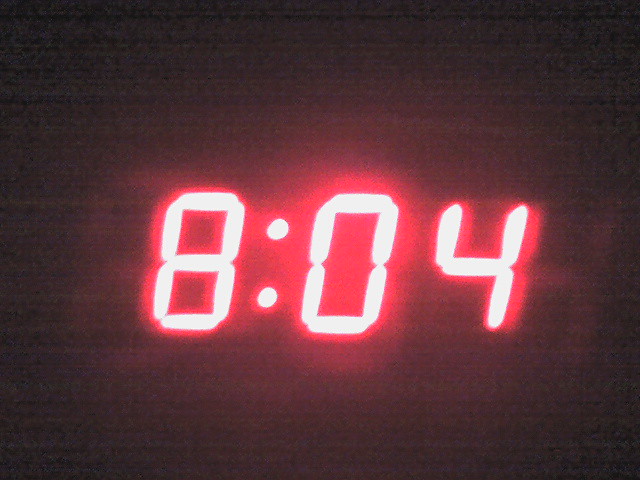The close-up image features the digital display of a clock, set against a black, horizontally lined background indicative of an LCD screen. The time, prominently displayed in the center, reads 8:04. The digits, rendered in crisp white LED with a striking red outline, exhibit a ghosting 3D effect; the red border appears to float behind the numbers, creating an illusion of depth. This intricate detailing suggests a meticulously captured moment, with the surrounding fuzziness highlighting the lesser resolution common in photographed screens. The ambiguous lighting leaves uncertain whether the time is 8:04 AM or PM.